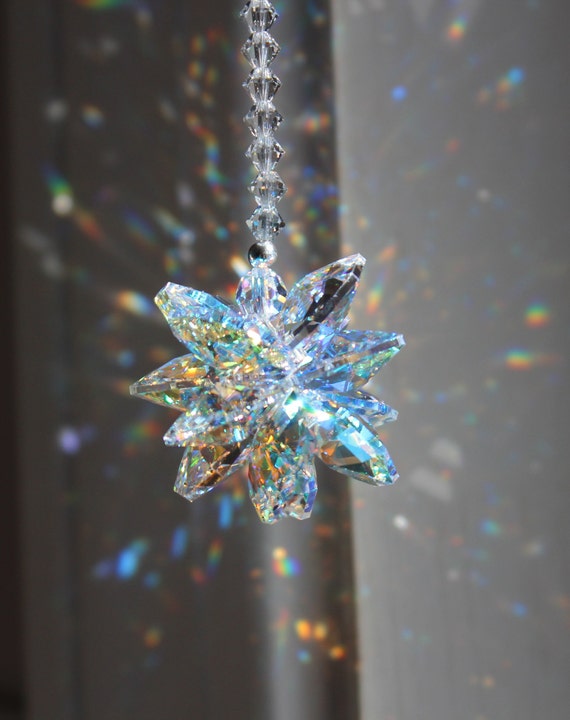This color photograph features a stunning crystal pendant with an abstract, faceted design resembling a decahedron or starburst with numerous points. The pendant is intricately detailed with multiple angled sections that create a textured, overlapping star shape. Suspended from a crystal string adorned with small, circular beads, the pendant emits brilliant, scattered rays of multicolored light—blue, orange, green, and more—creating a dazzling rainbow effect on the light gray background wall. The overall scene evokes the aesthetic of a high-quality product photo you might find on platforms like Etsy, Amazon, or Shein, capturing the crystal's luminous beauty and intricate design in a captivating, elegant manner.